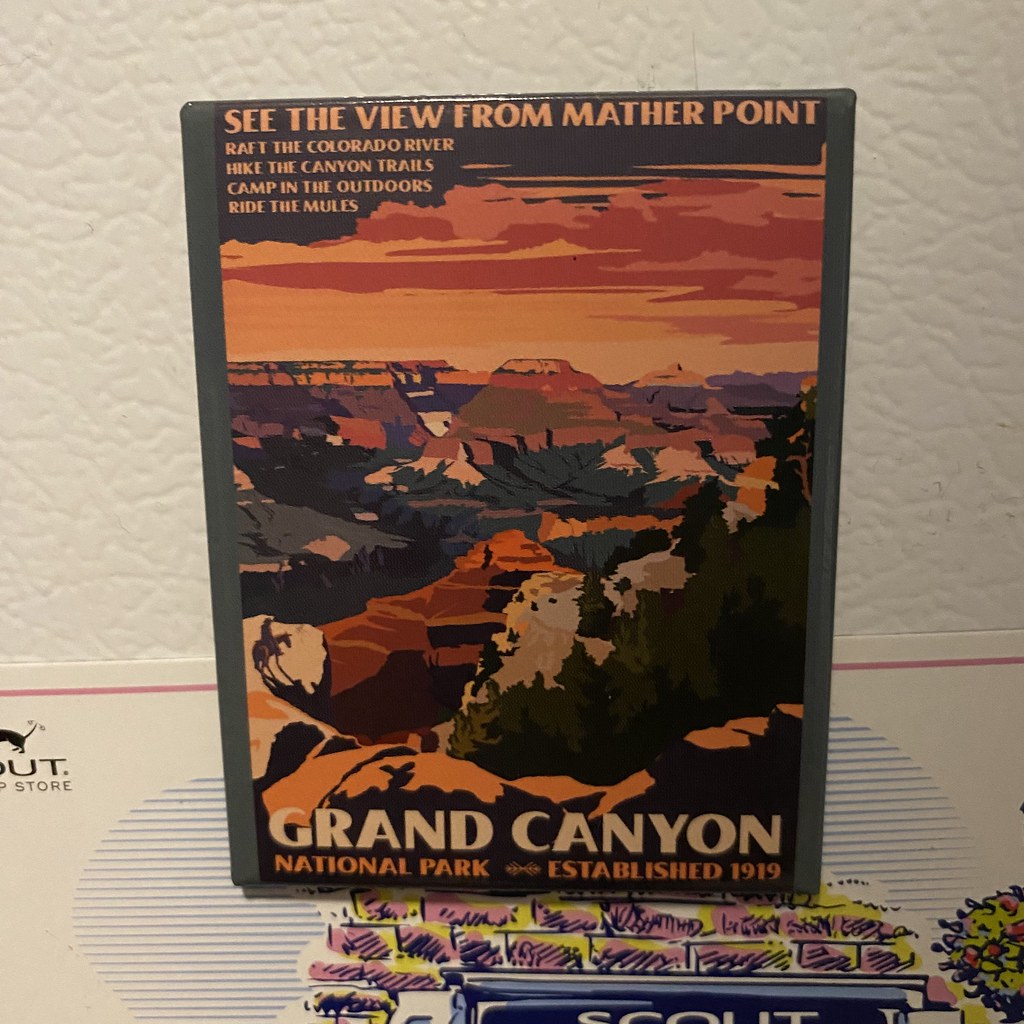This image features an advertisement poster for the Grand Canyon National Park. The poster stands against a white, textured wall and appears to be mounted on a surface with a gray backing or a mat with various symbols and abstract designs in blue, pink, and yellow. The top of the poster prominently displays the text "SEE THE VIEW FROM MATHER POINT" in bold, uppercase orange letters. Below this, four lines of orange text list activities: "raft the Colorado River," "hike the canyon trails," "camp in the outdoors," and "ride the mules." Dominating the poster's center is a stylized, abstract illustration of the Grand Canyon, painted in hues of orange, purple, gray, red, green, and blue, creating a vivid, almost cartoon-like depiction of the iconic landscape. The image includes detailed peaks and valleys, with a notable figure on horseback situated near the edge of a cliff, gazing over the expansive canyon. At the bottom, "GRAND CANYON" is written in large, white uppercase letters, with "National Park established 1919" in smaller, orange text beneath it.